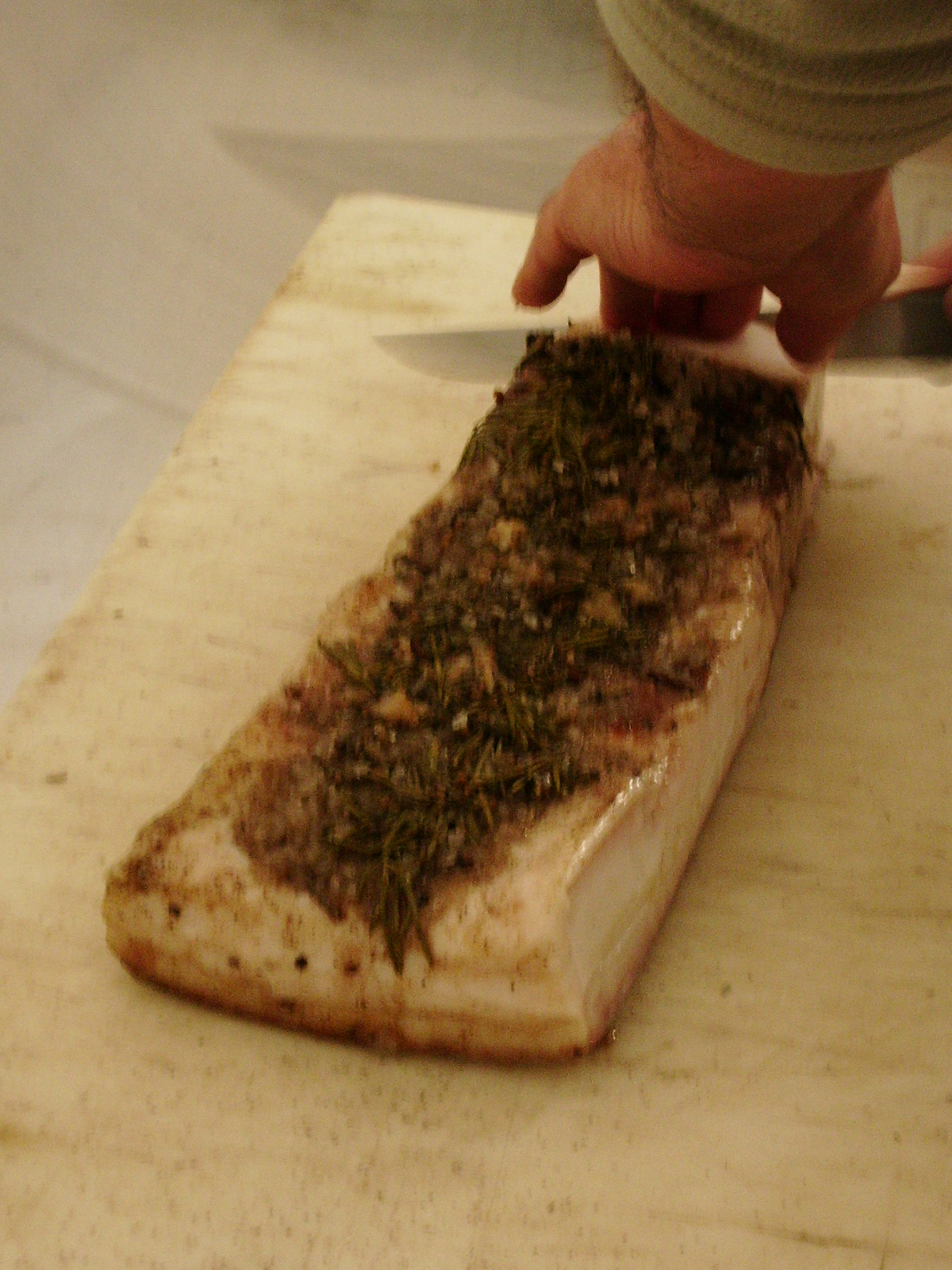In the image, a slightly hairy left hand and wrist extend from the upper right corner, partially obscured by the white cuff of a sweater. The hand is guiding a knife, cutting into a rectangular food item situated on a light-colored surface, possibly a cutting board. The item, which measures approximately a foot long and five inches wide, appears to be a piece of French bread with various seasonings and herbs scattered on top. The bread looks to have toppings that might be meat or cheese. The action captured in the frame shows the hand in the motion of slicing the bread into roughly one-centimeter-wide pieces.